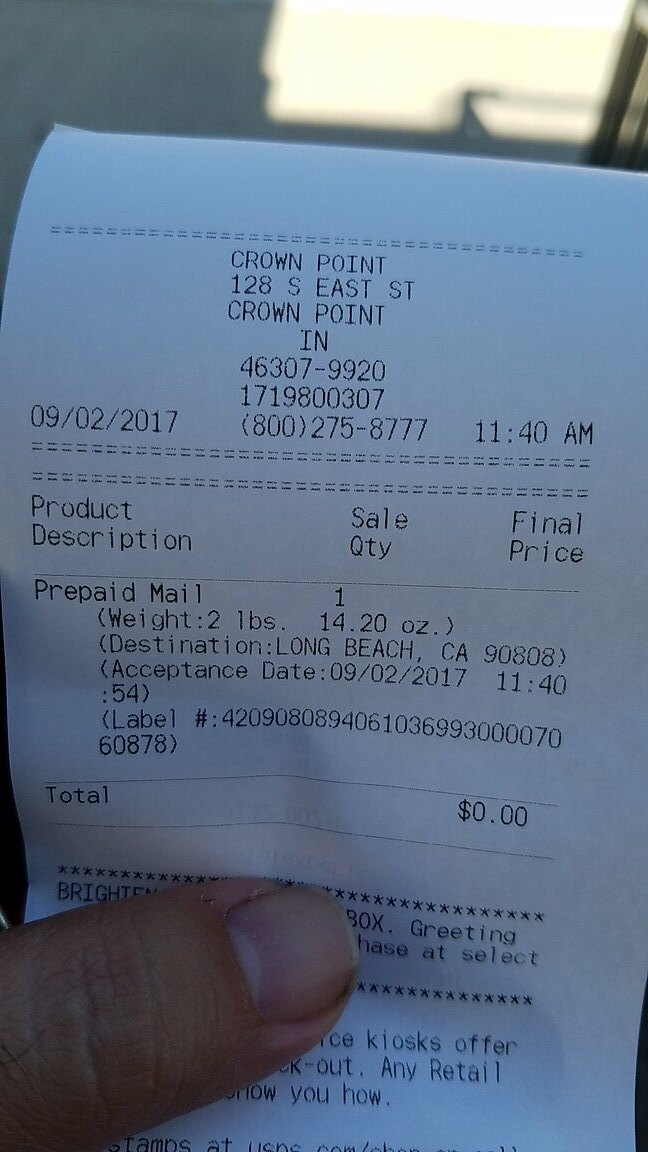A photograph captures an individual holding a white receipt with their thumb visible near the bottom of the image. The receipt prominently displays detailed information, including the address "128 Southeast Street, Crown Point, Indiana, 46307-9920" and a date of "September 2nd, 2017." It also shows the time "11:30 AM" and a phone number "1-800-275-8777." The receipt is for a prepaid mail item weighing 2 pounds and 14.2 ounces, with a destination of Long Beach, California. The final total on the receipt is $0.00, indicating it was prepaid. At the top of the image, behind the receipt, there's a faint glimpse of sunlight and shadow, highlighting that the photo was taken outdoors.